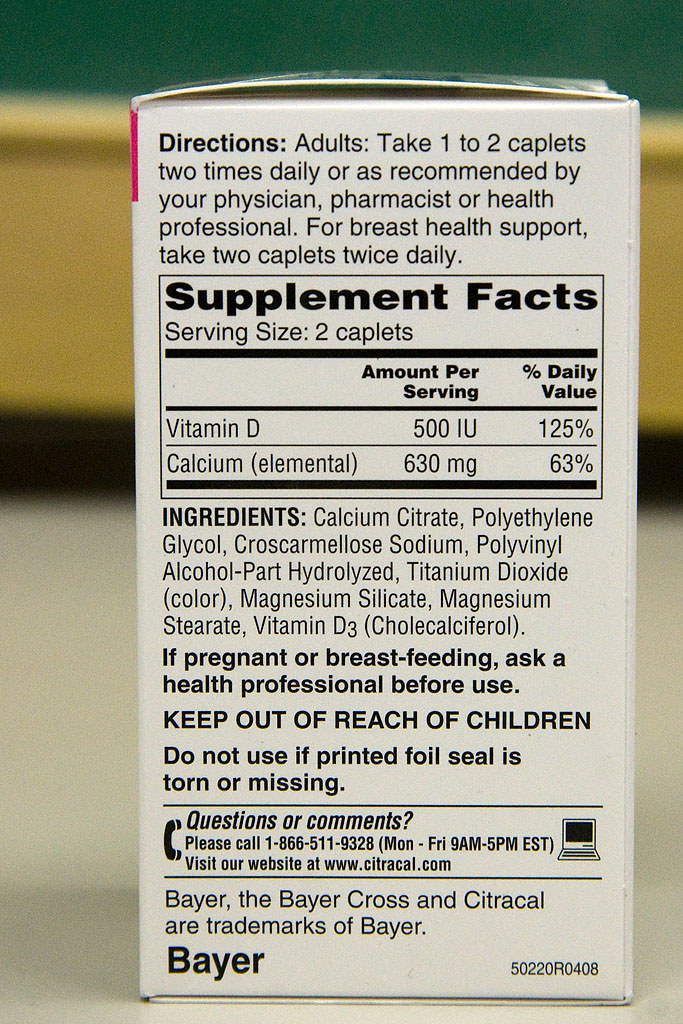The image depicts a side view of a white Bayer product box, likely a vitamin D and calcium supplement. The top features a small green stripe, followed by a wide yellow-white border, and a thinner brown border beneath. The box lid, made of cardboard, is slightly ajar at the top. In the top left corner, a prominent pink strip indicates where it says "Directions."

Below the directions, a black-bordered rectangle encloses the "Supplement Facts," detailing that each serving size is two caplets, providing 500 IUs of Vitamin D (125% of the daily value) and 630 mg of elemental calcium (63% of the daily value). Ingredients listed include calcium citrate, polyethylene glycol, cross-carmellose sodium, polyvinyl alcohol, partially hydrolyzed, titanium dioxide, magnesium silicate, magnesium stearate, and Vitamin D3.

Further down, bold black text states "Ingredients," followed by a list of the components and a warning: "If pregnant or breastfeeding, consult a health professional before use. Keep out of reach of children. Do not use if printed foil seal is torn or missing." Instructions also prompt for more information via a designated area to call or write to the company.

At the bottom left, in large bold letters, is the Bayer logo alongside the Bayer Cross. It also mentions that "Citracal" and "Bayer" are trademarks of Bayer.